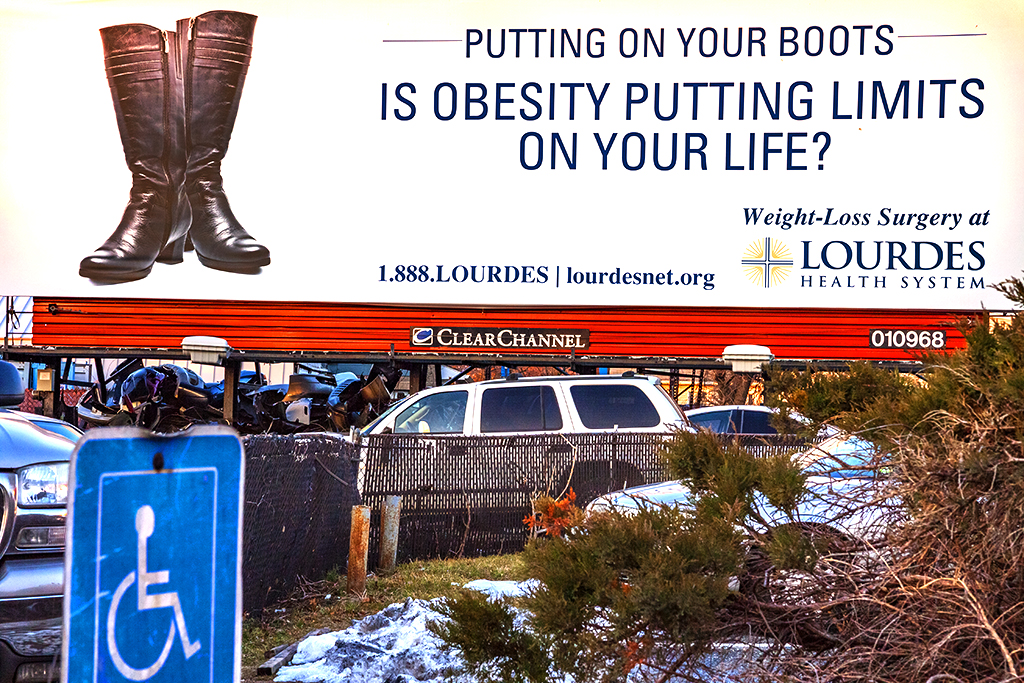The outdoor photograph features a billboard prominently placed at the top of the image. The billboard has a red base with the identifier "Clear Channel 010968." The main advertisement on the billboard is set against a white background and showcases a pair of tall, brown boots on the left side. The text on the billboard reads: "Putting on your boots is obesity putting limits on your life. 1-888-LORDSNET.org. Weight Loss Surgery at Lourdes Health System."

Below the billboard, the scene transitions to a green, grassy area interspersed with brown and green bushes, lightly dusted with patches of snow. Towards the bottom of the image, several cars, including a couple of white ones and a silver one, are parked in a parking lot. In the bottom left-hand corner, there is a partially visible blue sign with a white border, featuring a handicapped logo, indicating designated handicapped parking spaces.